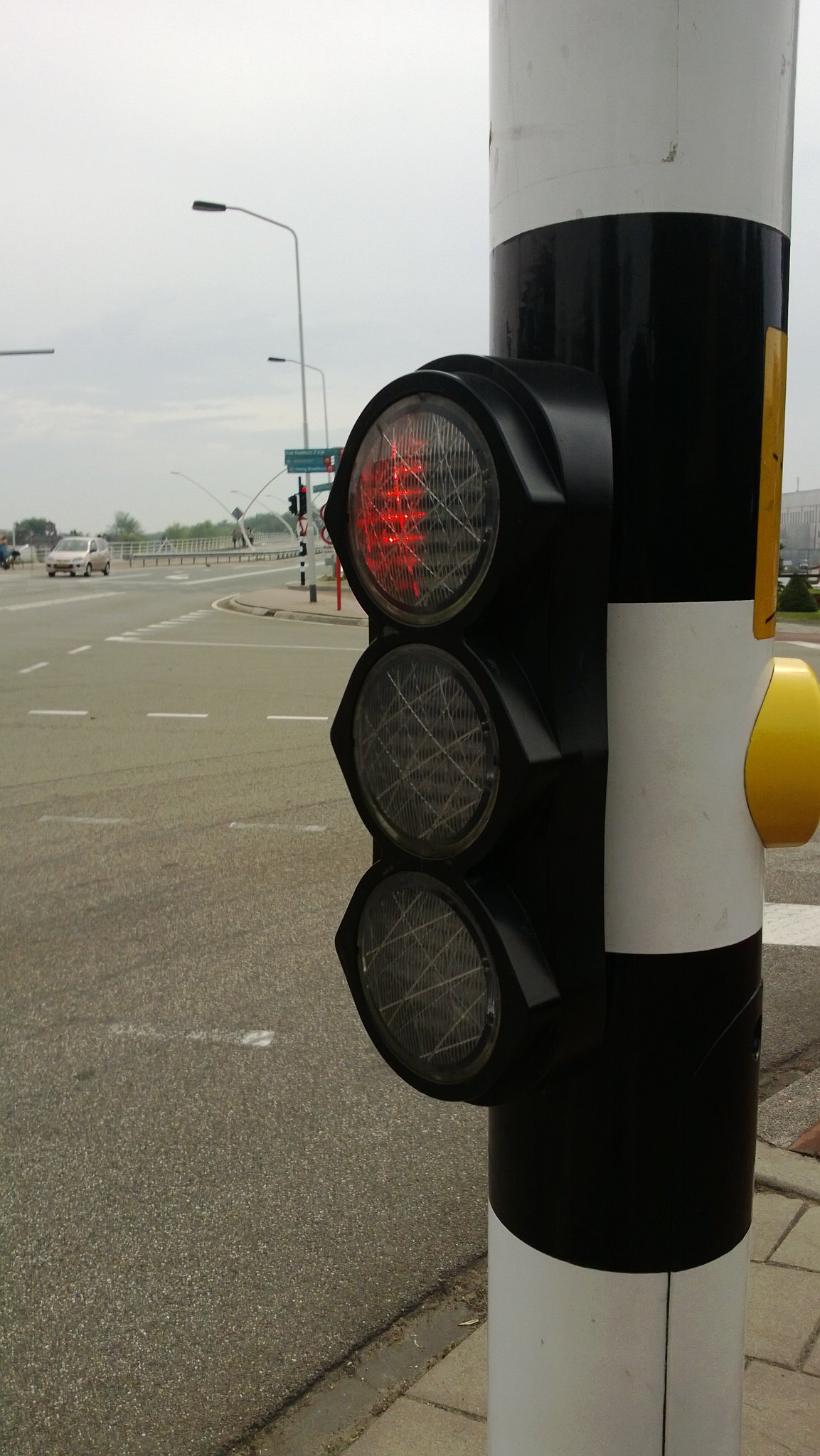This is a detailed color photograph of a pedestrian crosswalk signal on a major multi-lane road, possibly a boulevard or highway. Dominating the foreground, a large, round white pole with distinct black stripes supports a black traffic light box. The box houses three stacked circular lights, with the top one illuminated in red, though only partially; the middle and bottom lights remain unlit. Mounted unusually low at about two and a half feet from the base, the light is framed with a flush design, and lacks the typical hood. On the opposite side of the pole, there's a bright yellow button to activate the pedestrian crossing signal. 

Background details include an expansive asphalt roadway marked with white crosswalk lines and a distant vehicle. The scene's far end reveals tall streetlamps, green highway signs, and a steel guardrail, indicating a large, possibly urban intersection. The sky above is a mix of gray with hints of blue and light white clouds. The sidewalk at the base of the pole consists of paving stones, adding texture to the scene. The photograph captures a functional yet detailed urban infrastructure setup.